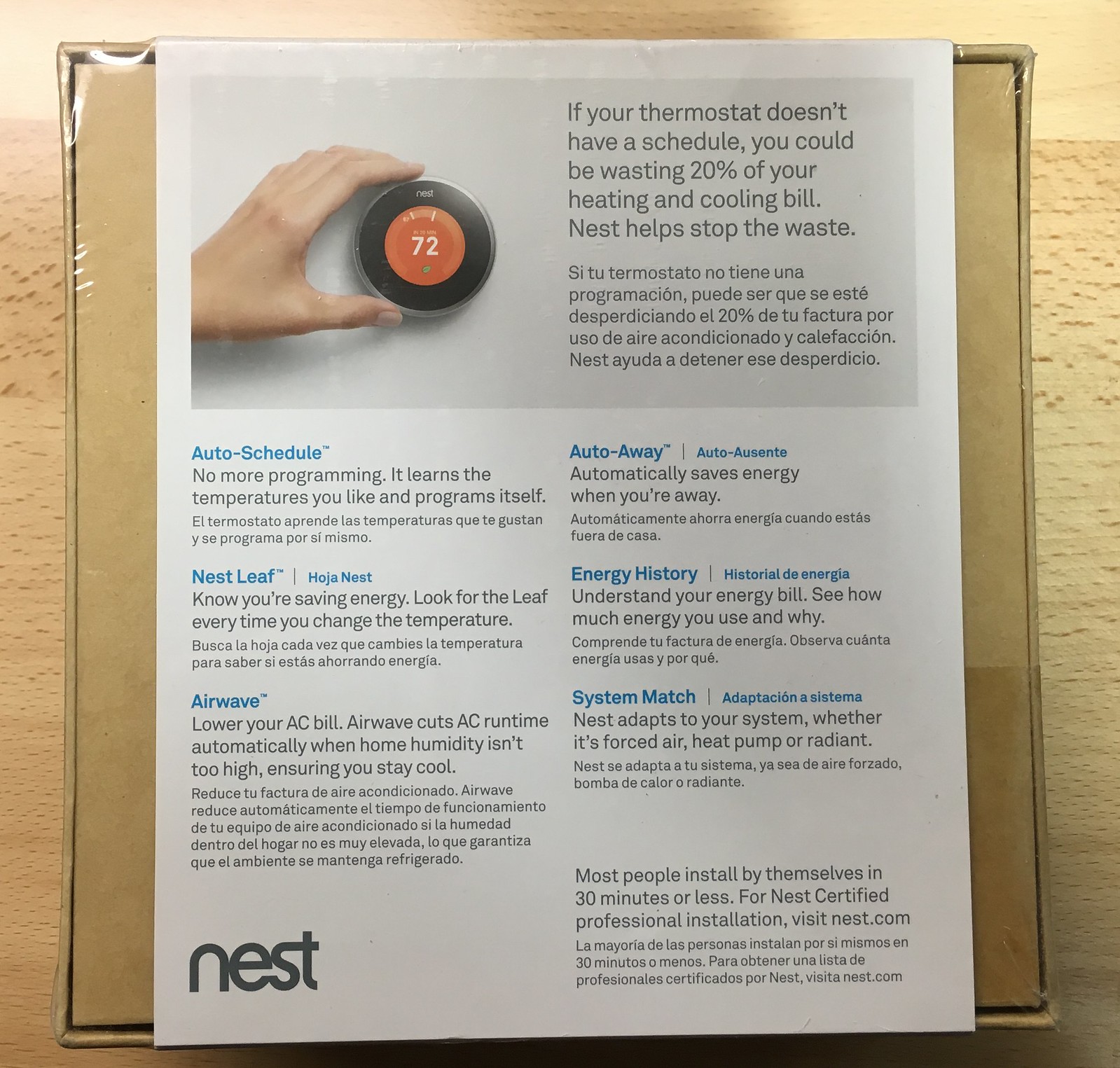The image features a white table as the background. Prominently placed on the table is a cardboard box wrapped in plastic, containing a prominently displayed page. On the top right of this page, there is a large gray square with text that reads, "If your thermostat doesn't have a schedule, you could be wasting 20% of your heating and cooling bill."

To the left of the image, a hand is shown interacting with what appears to be a Nest thermostat. The thermostat itself is designed with a circular interface. Surrounding the top of the circle, the word "Nest" is clearly displayed. The middle of the thermostat is highlighted in orange with a large white number "72" indicating the current temperature setting. The outer edge of the thermostat features a dial indicating a range from zero upwards.

At the bottom of the image, there is detailed text in blue, promoting various features of the Nest thermostat. It reads:

- "Auto-Schedule: No more programming. The thermostat learns the temperatures you like to program itself, ensuring energy savings and comfort. 
- Airwave: Lowers your AC bill. Airwave cuts AC runtime to 110% automatically when humidity isn’t too high, ensuring you stay cool.
- Auto-Away: Automatically saves energy when you're away.
- Energy History: Understand your energy bill. See how much energy you use and why.
- Nest Compatibility: Matches your system, whether it’s a heat pump or radiant. Most people install it in 30 minutes or less."

At the bottom left corner of the page, the word "Nest" is prominently displayed in bold black text.